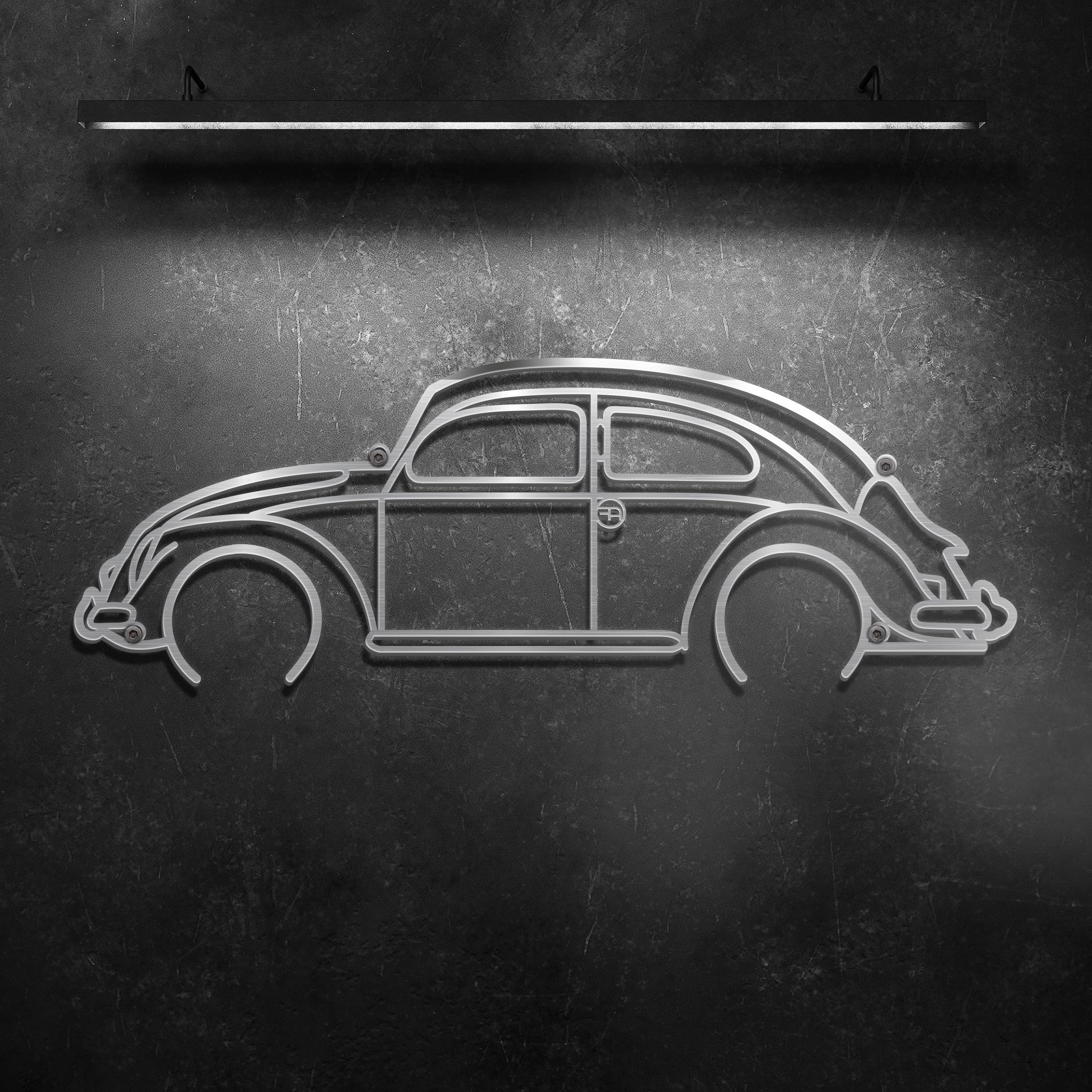The image shows a square, 6x6-inch, black and white photograph featuring a stylized wall-mounted relief sculpture of a classic 1970s Volkswagen Beetle, or VW Bug. The sculpture itself is crafted from a single sheet of material, likely brushed stainless steel or possibly extruded plastic, and presents an elegant outline drawing of the Beetle. This detailed outline includes the windows, doors, fenders, headlights, and bumpers, with the wheels distinctively open at the bottom. The sculpture is set against a dark gray, textured slate wall. The wall has light gray scratches, adding texture to the background. Above the sculpture is a thin, horizontal light fixture, held by two bars on either side, which casts a soft illumination down onto the Beetle, creating a subtle drop shadow and highlighting its reflective surface. The front of the Beetle is oriented to the left, with its unmistakable shape clearly represented in the minimalistic, yet detailed art piece.